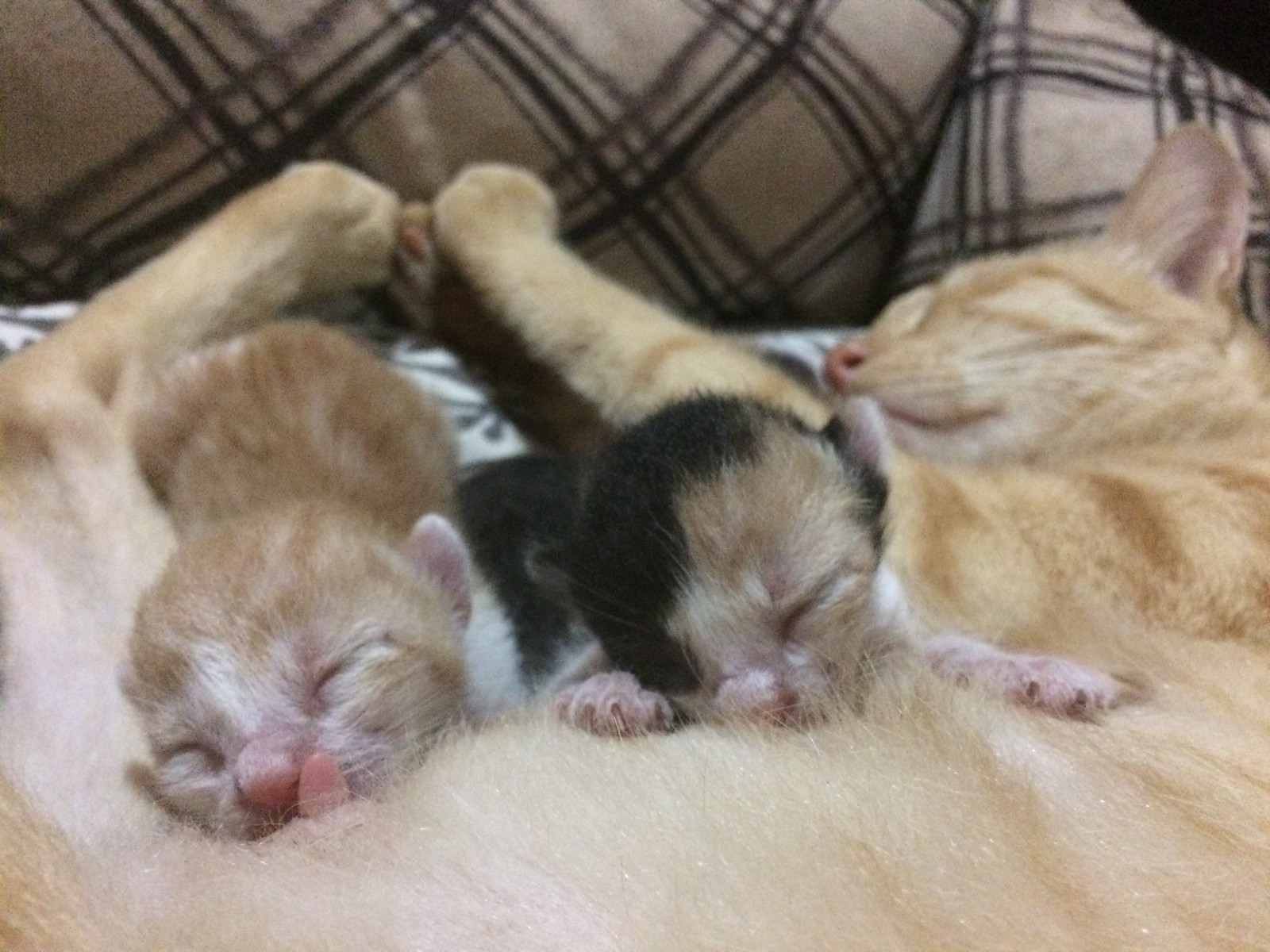In this image, a mother cat and her two kittens are peacefully resting on a soft, plaid-patterned cat bed that features a mix of brown, black, and white colors. The mother cat, a light brown tabby with a pink nose, is curled up and fast asleep, her feet extended towards the top of the picture. Her eyes are gently closed as she provides a comfortable spot for her kittens. The kitten on the right, positioned to the left of the picture, has a striking fur pattern with a black and brown face and closed eyes as it kneads its mother for milk. The other kitten on the left closely resembles its mother with a similar light brown tabby coat and a pink nose. Both kittens are nestled close to their mother's stomach, evidently trying to feed. The overall setting appears to be indoors, and aside from the cats, there's no visible text, just a cozy scene of a feline family in a serene moment of bonding.